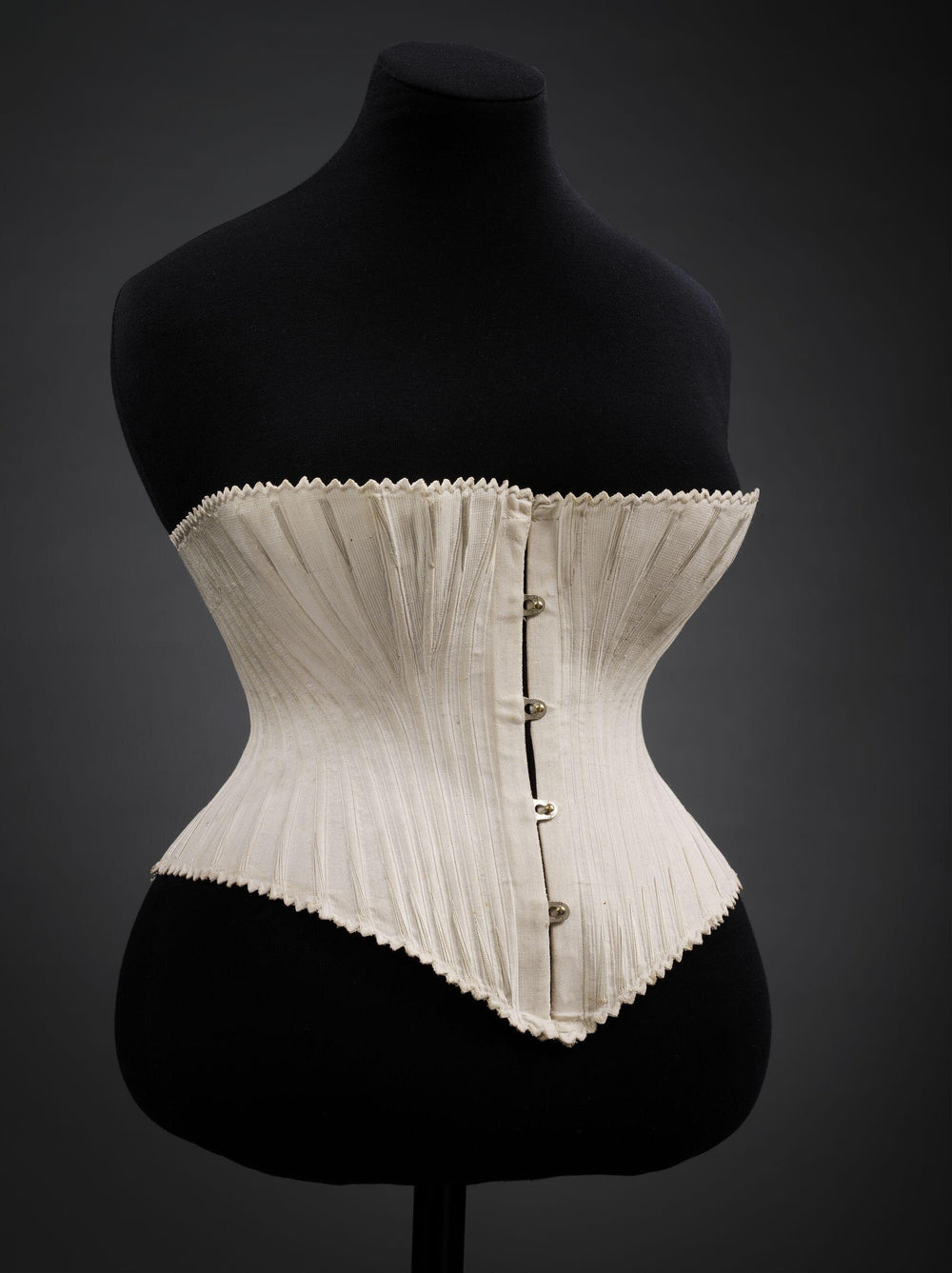The photograph showcases a detailed, Victorian-inspired corset worn by a black torso mannequin with no head, arms, or legs. The corset is a delicate cream or beige color with four prominent green buttons down the front, and it fits the mannequin's form closely, extending from just under the bust to below the belly button. The fabric features subtle vertical textures and intricate Victorian details, including scalloped edges at the top and bottom that resemble a picket fence. Additionally, there are silver hooks for closure that run down the middle. The mannequin stands against a dark gray background that lightens subtly towards the center, enhancing the vintage, artistic appeal of the image.